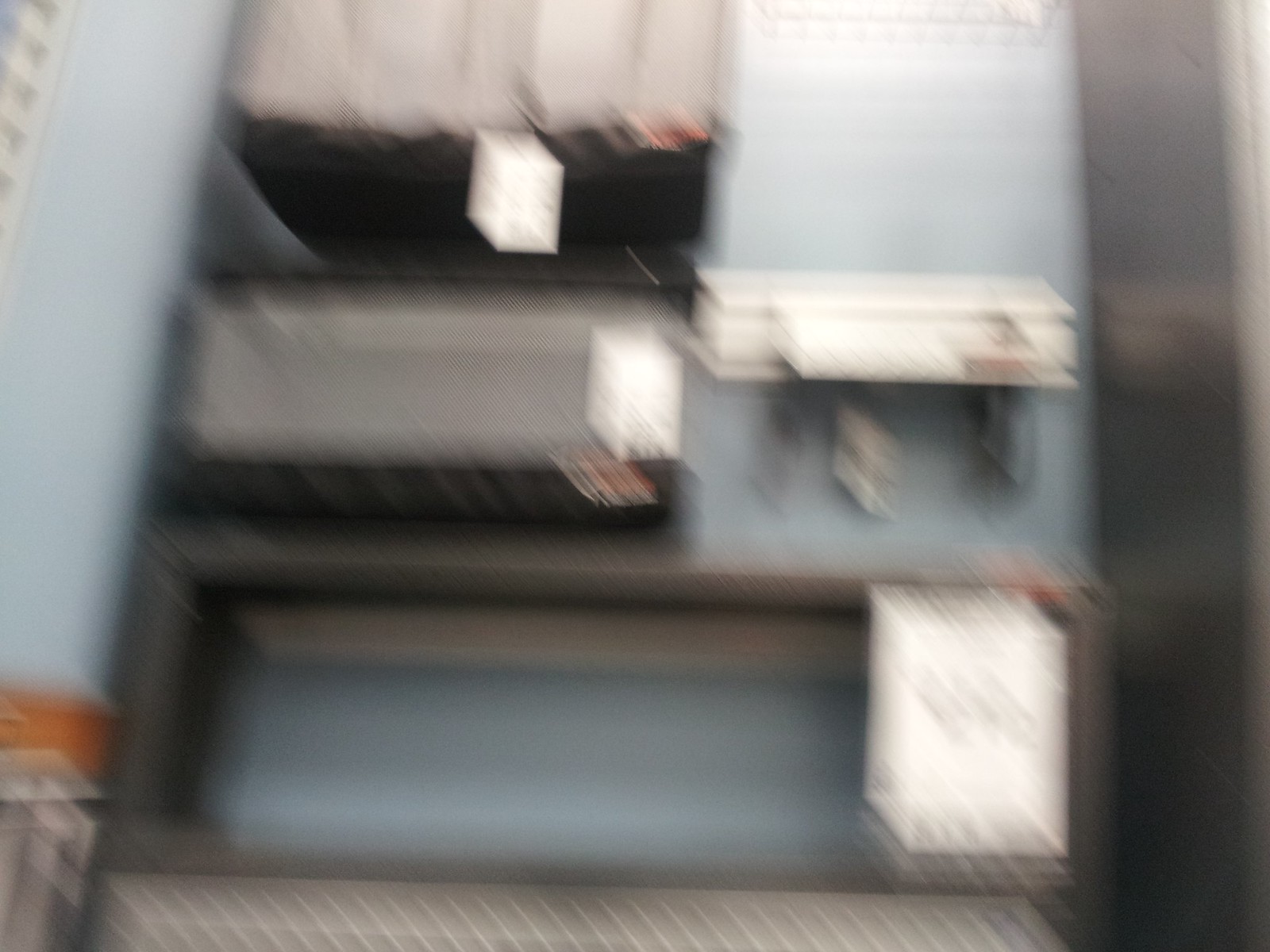In this highly blurred image, it is challenging to discern the precise subject matter. The predominant color is a soft light blue, which envelops the scene entirely. A light cream pattern extends horizontally across the bottom region of the image. To the right of this cream section, there is a white rectangle on the left-hand side, encircled by a brown border. Above the central area, there appear to be additional items or structures, potentially files or containers, though the extreme blurriness makes their identification difficult. The light blue hue continues to frame the image on all sides.